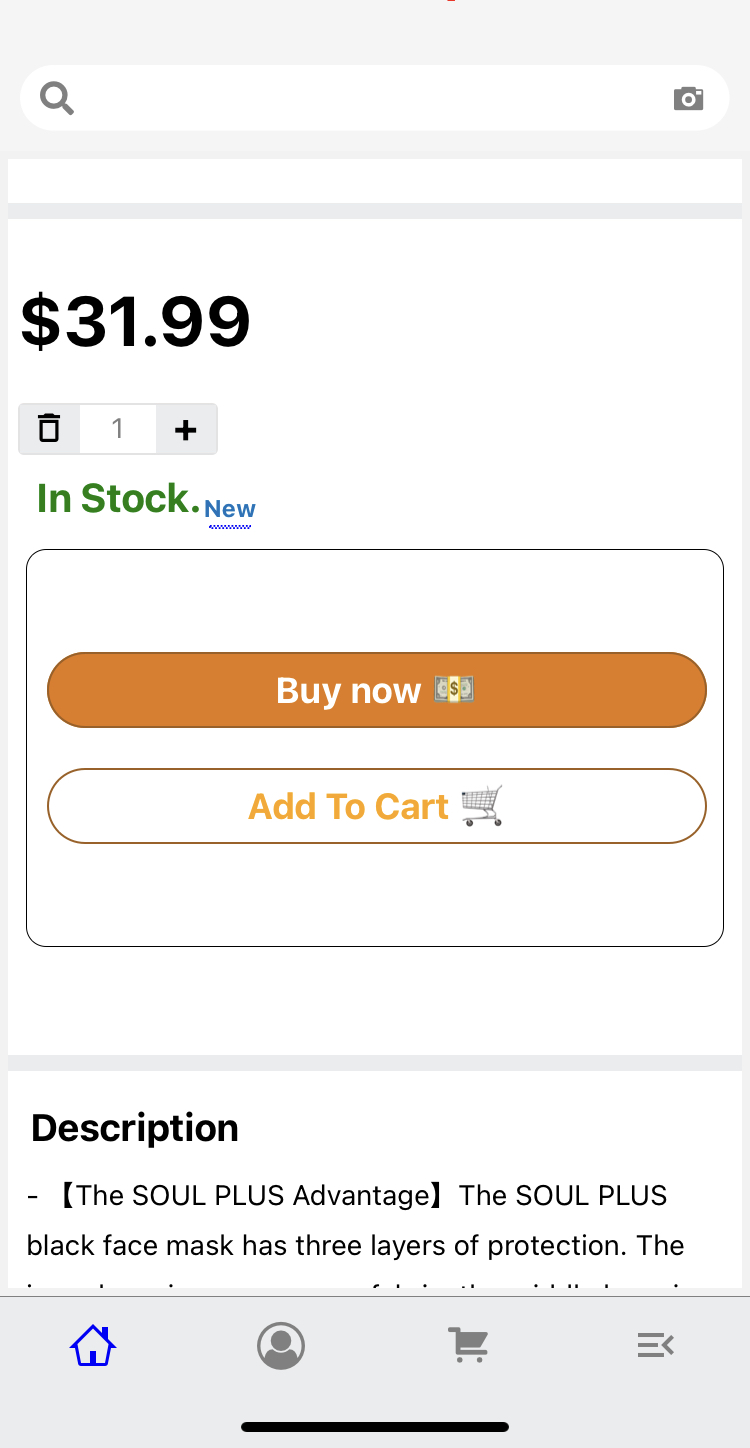This is a detailed and cleaned-up caption for the described image:

---

The image is a portrait-mode screenshot featuring a predominantly white background. At the top, there's a search bar with no text entered. Below the search bar, in bold black font, the price "$31.99" is prominently displayed. Beneath the price, the text "In Stock" is written in green, while "New" is indicated in blue. 

The following section contains two buttons: a large orange "Buy Now" button with a small-font image of a US dollar next to it, and a large clear "Add to Cart" button that includes an icon of a shopping cart. The text on both buttons is smaller than the buttons' size, leaving much unused space.

Further down, in bold black font, the word "Description" is followed by "(The Soul Plus Advantage)," indicating additional product information. The description begins with "The Soul Plus Black Face Mask has three layers of protection. Then the..." before being abruptly cut off, possibly due to the user scrolling down further.

The overall context suggests that the product being considered for purchase at $31.99 is the "Soul Plus Advantage Black Face Mask," with no indication of quantity provided in the visible portion of the screenshot.

---